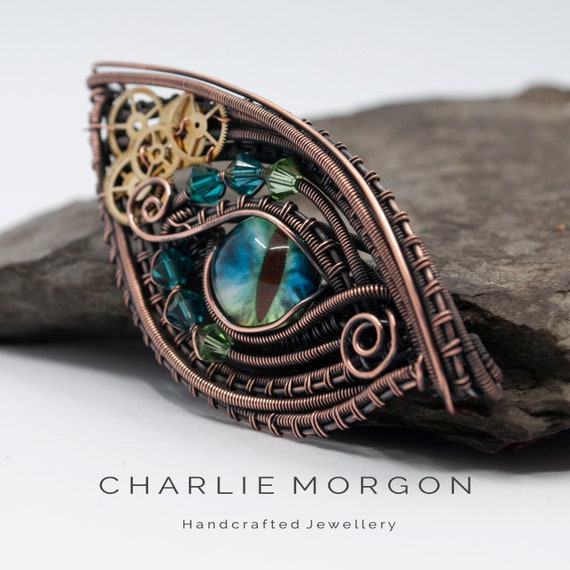The image showcases a distinctive and handcrafted piece of jewelry by Charlie Morgan, prominently advertised as "Charlie Morgan Handcrafted Jewelry" at the bottom. The central piece of the jewelry is an intricately designed ring or pin shaped like an eye, exuding a steampunk aesthetic with an Egyptian flair.

The eye-shaped jewelry features a captivating, vertical iris resembling a cat or snake eye, with a striking blue color complemented by dark blue and green streaks. Surrounding the eye are numerous details that add to its allure: several gold gears positioned around the narrow part of the eye, contributing to the steampunk look; and various gems, including two blue and one green stone, situated just above the eyelid.

Constructed from a darker copper or possibly rose gold metal, the piece has a rich bronze tone with metallic tubing forming the body. Twists, coils, and swirls of metal, particularly a prominent swirl on the bottom right side, enhance its unique appearance. Resting against what looks like flagstone rock, the jewelry's intricate design and color palette of bronze, gold, blue, and green create a visually striking and unusual accessory.